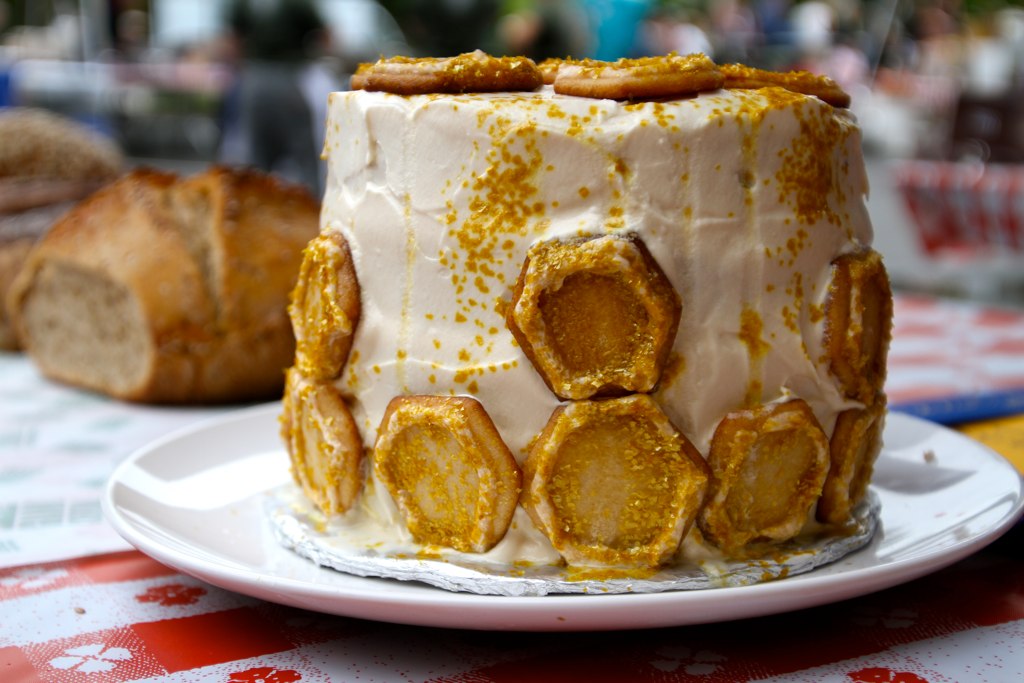In this brightly lit outdoor photograph, a round, layered dessert cake takes center stage on a white plate, which rests on a red and white checkered tablecloth. The cake is adorned with white frosting and decorated with golden, hexagon-shaped cookies that encircle the base in a solid ring, gradually becoming spaced out on the upper layers. The top of the cake features additional brown cookies and colorful confetti-like sprinkles. In the background, a partially sliced loaf of whole grain or sourdough bread is visible. The image appears to capture a celebratory scene, perhaps a picnic or gathering, with other attendees blurred out to emphasize the cake as the focal point.